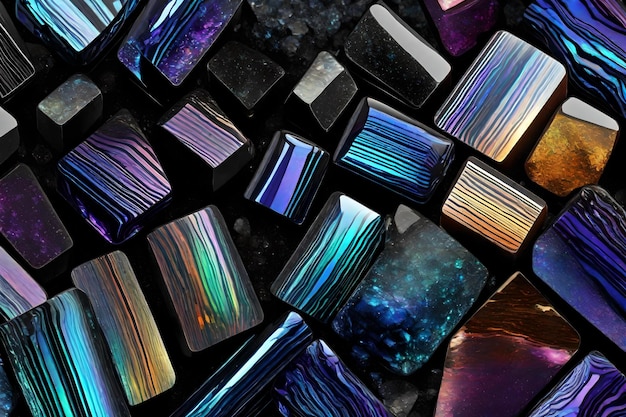This is a photograph of a collection of intricately cut stones, each with unique colors and patterns, meticulously laid out on a black surface. The image, taken in landscape orientation, captures approximately 20 to 25 stones of various shapes—primarily rectangular and square—arranged side by side yet facing different directions. Each stone exhibits distinct characteristics: some are purely monochromatic, while others are adorned with vibrant stripes and layers. You can find stones with dark blue and purple, pink with blue stripes, and multicolored stripes including green, pink, orange, and reddish hues. Other stones display shades of aqua, blue, and black, often with a shiny, metallic reflection that highlights their polished surfaces. These geometrically shaped stones, divided into smaller squares and rectangles, create a captivating mosaic of color and light across the rectangular frame of the photograph.